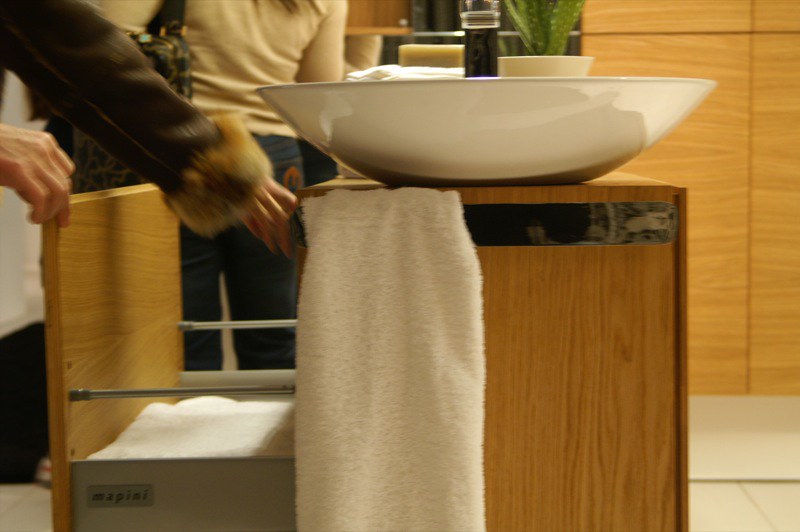A detailed photograph showcases an Asian-inspired kitchen or bathroom setting. The focal point is a side view of a brown wooden counter cabinet, which features both a bottom cabinet and a countertop. Atop the counter sits an exceptionally large, wide bowl, either made of white china or metal, hinting at its utility. Draped over the left-hand side of the counter is a white towel, extending vertically from the center to the bottom of the image. Adjacent to this towel, a drawer, also part of the wooden cabinet, is pulled out, revealing a neat stack of more white towels within this low-profile compartment.

The left side of the frame captures the right hand of an individual gripping the drawer's right corner edge. Simultaneously, a left hand, likely belonging to another person due to the heavy jacket with a fur-lined sleeve it dons, is interacting with the contents inside the drawer. Dominating the center background, the back of a person wearing a tan, wrinkled sweater or t-shirt is visible. Judging by the direction of the wrinkles, this individual appears to be reaching upward with their left hand, suggesting they are simultaneously reaching with their right arm, partially visible on the right side of the image. Finishing the scene, the upper right corner of the counter displays a small white bowl housing a succulent plant, adding a touch of greenery and life to the space.